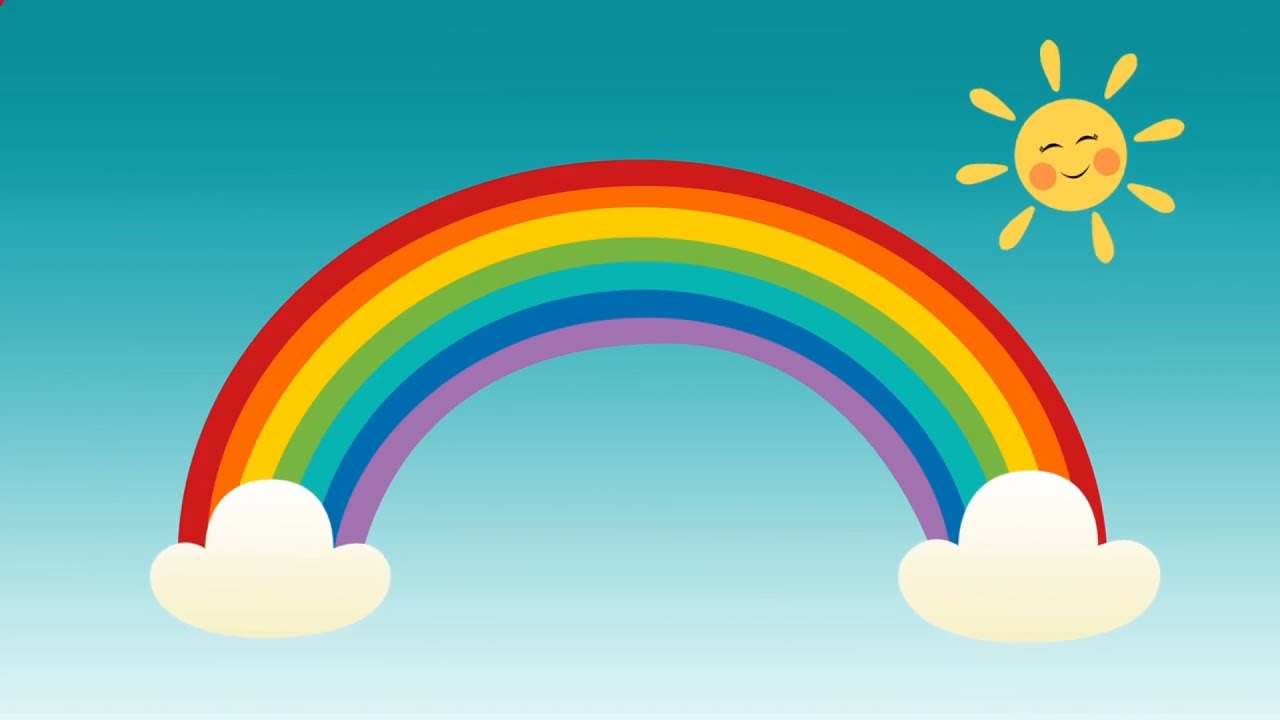The image features a whimsical, cartoon-like scene set against a graduated blue background, which transitions from a lighter blue at the bottom to a darker blue at the top. Dominating the center of the scene is a vibrant rainbow, flanked by identical, rounded clouds at both ends. The rainbow's colors, starting from its outermost band, are red, orange, yellow, green, light blue, dark blue, and purple. To the upper right corner of the image, a radiant sun with teardrop-shaped rays extends outward from its round, yellow body. The sun displays a cheerful face with two curved lines for eyes, an arched smile, and rosy orange cheeks, enhancing the overall joyful and child-friendly atmosphere of the artwork. There is no text present in the image.